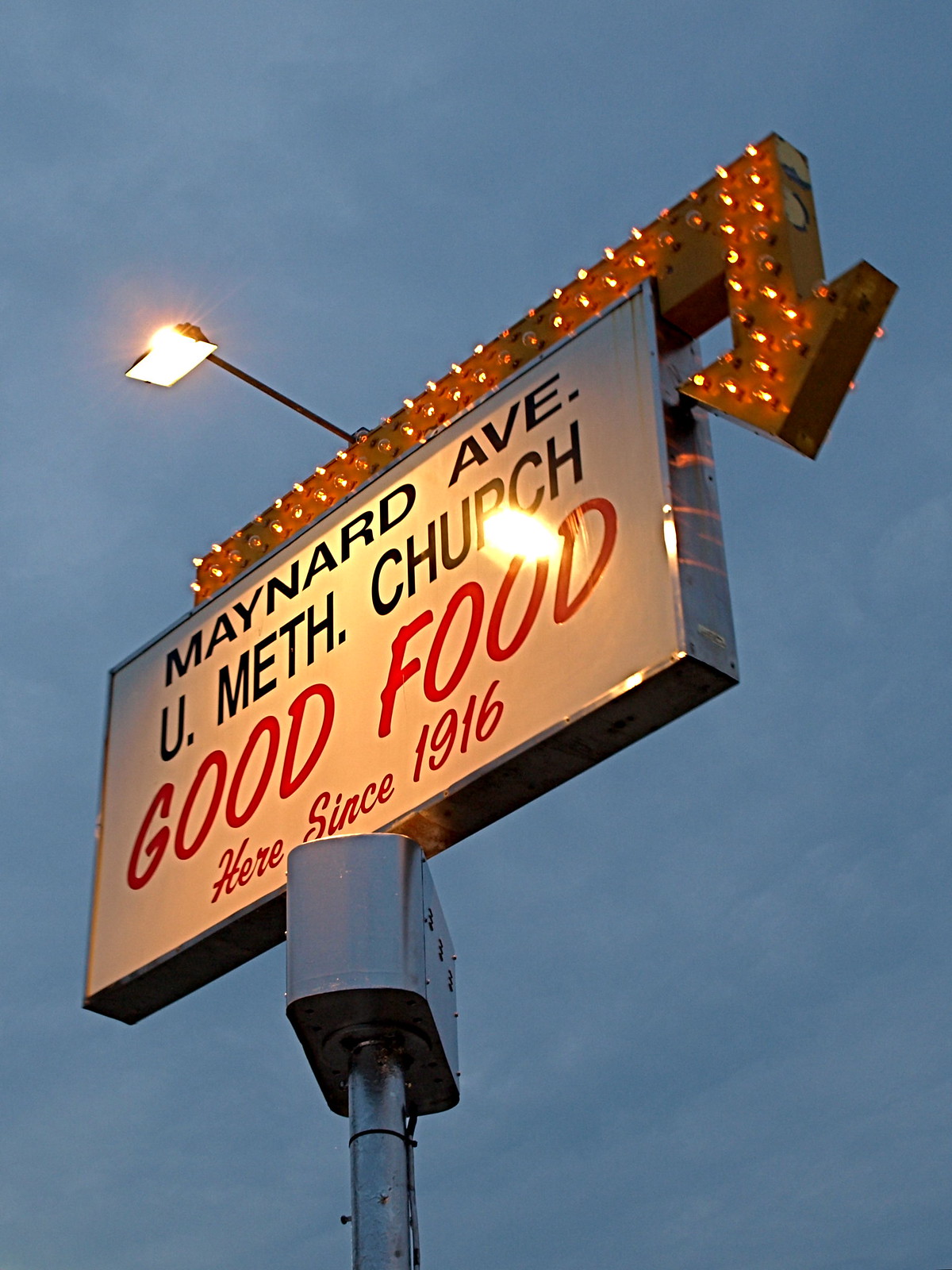The image features a large billboard sign positioned prominently against a dusky sky, characterized by a darker blue hue suggestive of approaching nightfall. The sign itself is supported by a silver-colored, sturdy metal pole, and the main focal point of the sign is a white rectangular panel with bold black and red lettering. In black font, the top part of the sign reads "Maynard Avenue, United Methodist Church," and directly beneath it, in striking red letters, it declares "Good Food Here Since 1916." 

Adding a dynamic element to the sign is a prominent arrow above it, extending horizontally from the left side, continuing above the sign, and then pointing downwards on the right. This arrow is adorned with numerous small, vibrant white lights, giving it a festive appearance. Enhancing visibility, a floodlight above the arrow casts illumination onto the sign below. The overarching scene is devoid of people, focusing entirely on the illuminated sign against the serene evening sky.